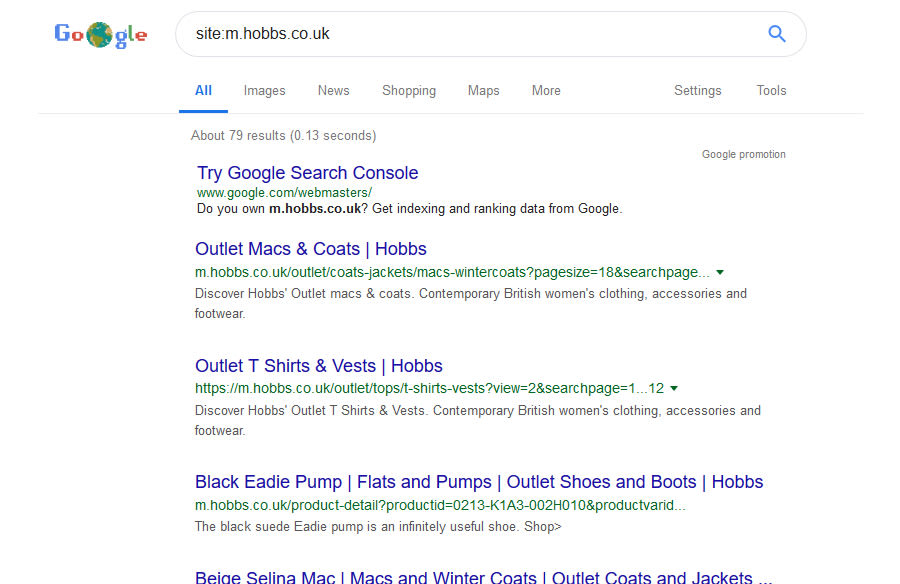Here is a detailed and cleaned-up caption for the given image:

---

The image displays a Google search results page for the query "site:hobbs.co.uk" focusing on the mobile version (m.hobbs.co.uk) of the Hobbs website. The search results highlight various categories from the Hobbs Outlet, including sections for "Outlet Mac & Coats," "Outlet T-Shirts & Vests," "Black & D-Pump," among other related items. These results underscore the availability of a wide range of clothing items and accessories from the Hobbs Outlet. The page predominantly features a clean, white background with blue and black text, characteristic of standard Google search interfaces. At the top of the page, there are navigation links near the search bar, facilitating easy access.

---

This caption captures the essence of the search results while adding a layer of specificity and structure.